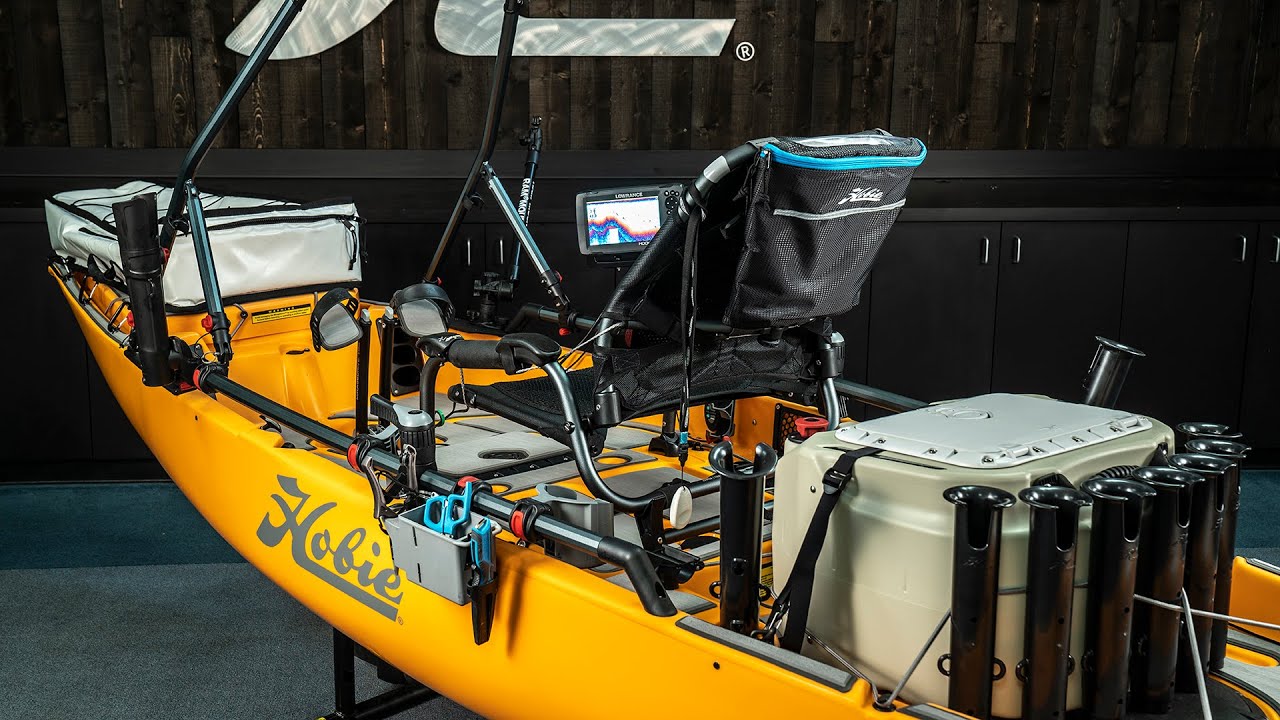This color photograph captures a detailed indoor scene featuring a kayak. The kayak, prominently displayed on a black stand, is placed within a building adorned with wooden walls and black cabinets with silver handles along the bottom. The kayak itself is primarily orange and gray, with the brand name "Hobie" inscribed in gray cursive on the side. At the rear, a tied-down box is positioned, surrounded by several black cylinders, while a black chair equipped with a GPS system occupies the middle. The front end of the kayak, facing the upper left portion of the image, features a white vinyl pack. The setting includes a concrete floor, further emphasizing the indoor environment.